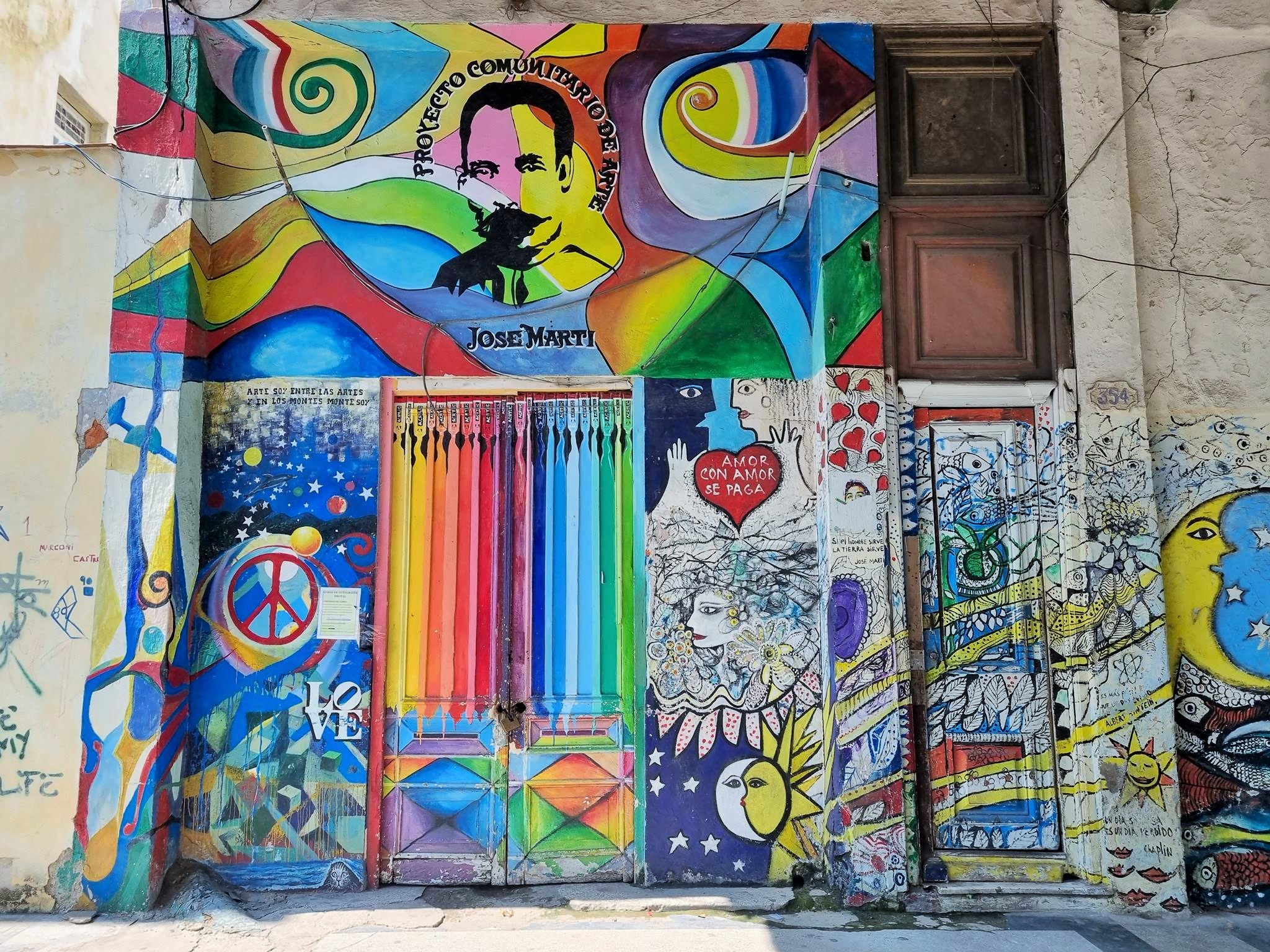The image depicts the side of a public building in a Spanish-speaking country, possibly in a lower-end part of town, adorned with an expansive, colorful display of artistic graffiti. At the center of the mural, prominently featured, is the face of Jose Marti, along with his name and possibly a motto in Spanish above him. Surrounding his portrait is a vibrant array of artwork including a peace sign, a crescent moon with stars, a sun illustrated with dynamic rays, and flowers. Additional imagery includes a woman's face, hearts, fish, and other intricate modern designs, some of which are line drawings yet to be colored in. Despite the building's dated and stained exterior, the mural transforms it into a captivating canvas of multi-colored expressions, encouraging viewers to revisit and discover new details with each glance.